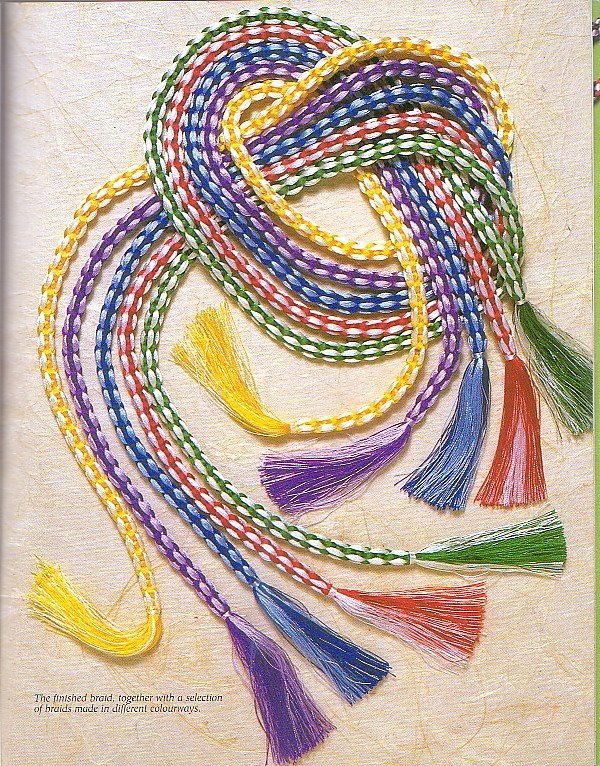This promotional product photo showcases an artistic arrangement of five braided ropes with corresponding tassels. Each braid features a combination of colors: yellow and white, purple and white, blue and white, red and white, and green and white. The ropes are intertwined to form a loose knot, displaying their vibrant colors against a cream-colored background. The tassels at the end of each rope add a decorative touch that complements the braided strands. A description at the bottom of the image reads, "the finished braid together with a selection of braids made in different colorways," indicating that this might be part of a catalog showcasing these colorful and intricately designed braids.